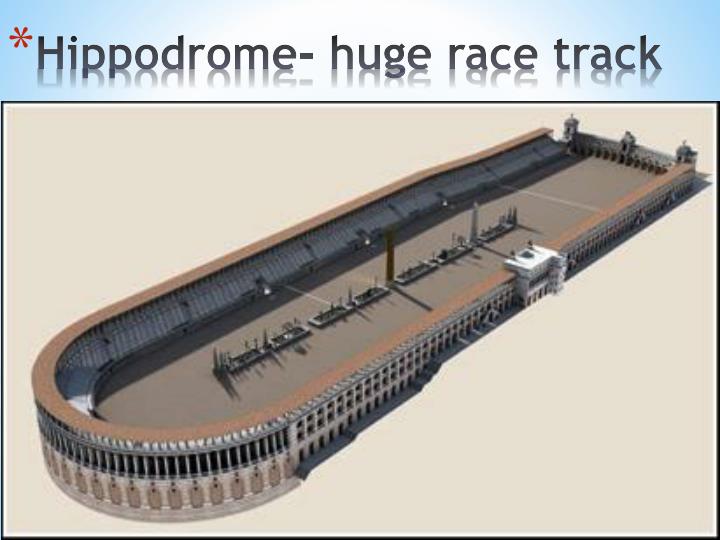This image is a detailed 3D rendering of a hippodrome, evoking the grandeur of ancient Roman architecture. At the top, there's a wide, thin rectangular bar with a gradient background that transitions from light blue on the sides to white in the center, reminiscent of a sky. Overlaid on this gradient is black text that reads "hippodrome - huge racetrack," with a red asterisk positioned above the capital "H" of "hippodrome." Below this header lies a larger horizontal rectangle bordered in black, containing the main visual of the hippodrome.

The racetrack itself is long and oval-shaped, framed by grand, coliseum-like architecture. The exterior of the building appears beige or light brown, with a brown-tiled roof. Surrounding the track is multi-story stadium seating, marked by numerous pillars and arches that emphasize its ancient style. The interior features several islands adorned with monoliths and greenery, around which the track loops in an elongated oval. The ground of the racetrack is a dusty grey or brown, adding to the historic and timeworn ambiance of the scene.